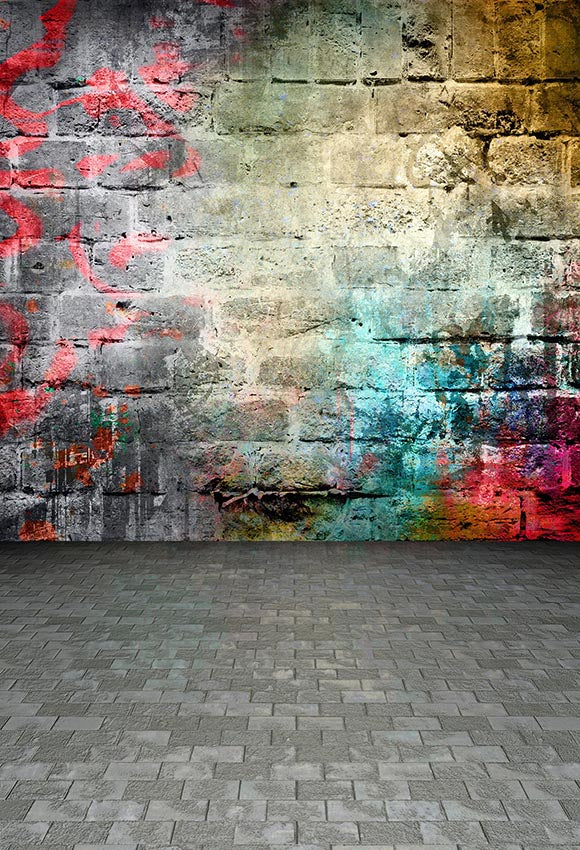The photograph captures a brick wall with a brick sidewalk leading up to it. The sidewalk is composed of square, gray bricks, creating a modern tiled look in front of the older, graffitied wall. The brick wall, which appears to be undergoing graffiti removal, displays a variety of paint colors. The central area of the wall looks like it has been power washed, leaving it bare compared to the colorful surroundings. To the left of this clean section, remnants of red paint and barely recognizable writing are visible. The right side features more multicolored paint splatters, including shades of cyan, pink, yellow, purple, and red, though this area also seems less vibrant, possibly a result of an earlier cleaning attempt. A standard drain hole is embedded into the brick near the bottom. Ambient lighting, likely from an overhead source, illuminates the scene, casting soft shadows and highlighting the textures of the aged, painted bricks. The overall impression is one of an urban environment caught between creative expression and restoration.